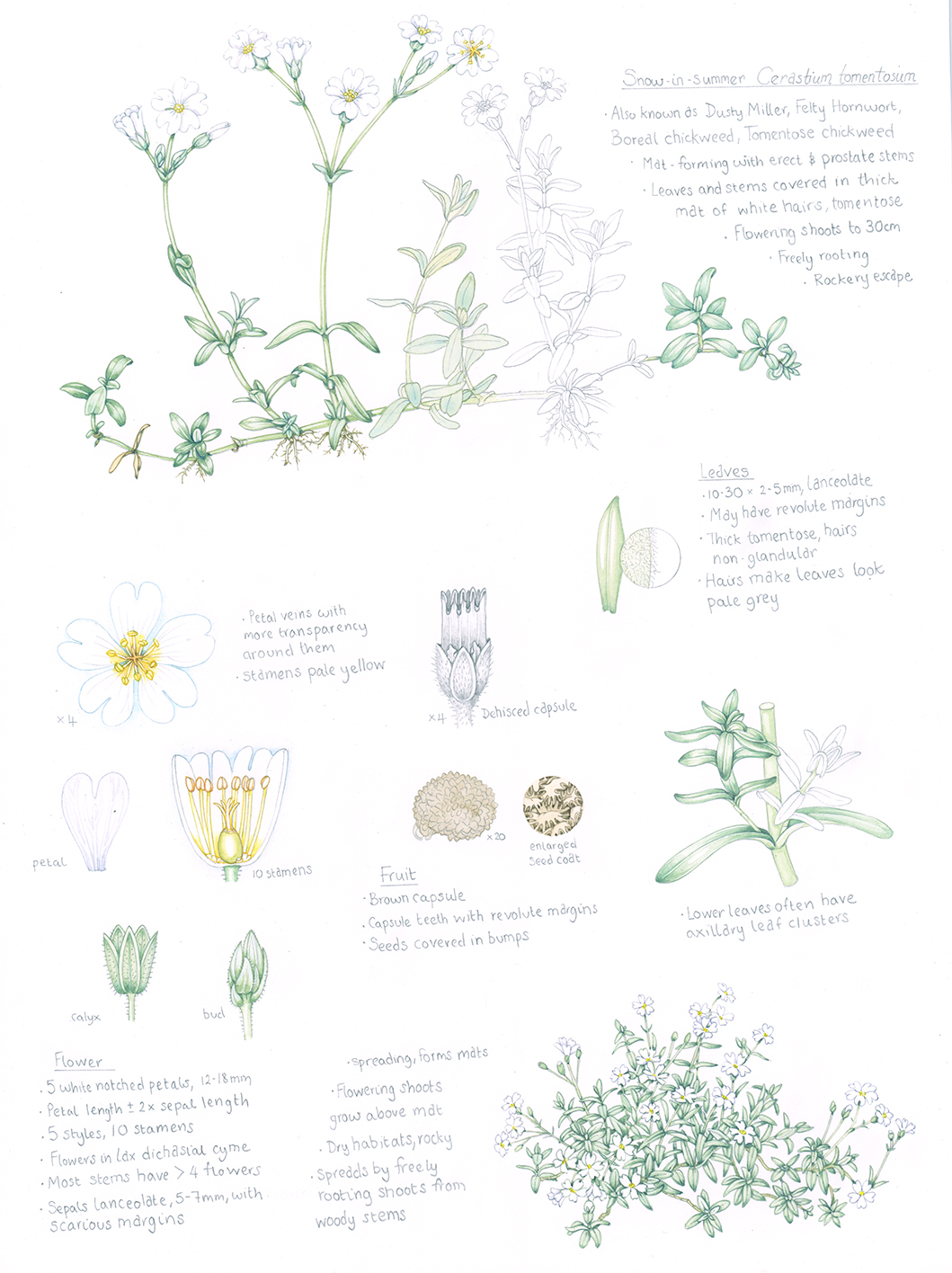The hand-drawn image appears to be a page from a flower or tree identification book, featuring detailed, color-painted illustrations and descriptions of different types of plants. At the top, there is a cluster of small, white flowers with yellow centers, about four or five on each branch. To the right, there is some writing, though it is too small to read clearly. Below this, a series of drawings depicts the stages of a flower opening, starting from a bud and progressing to a fully bloomed flower, each accompanied by text that is also difficult to decipher due to its size. The top right corner includes the names "Snow and Summer," also known as "Dusty Miller," as well as "Fighting Homewood" and "Born Chickweed." Lower on the right, additional names such as "Leadbees," "Mayhide," and "Revolut Merchants" are written. A white flower labeled "Petal Veins" is shown with some notes, and the bottom left features a green flower labeled simply "Flower." Finally, in the bottom right corner, there is another cluster of white flowers similar to those at the top, completing the detailed botanical illustration.